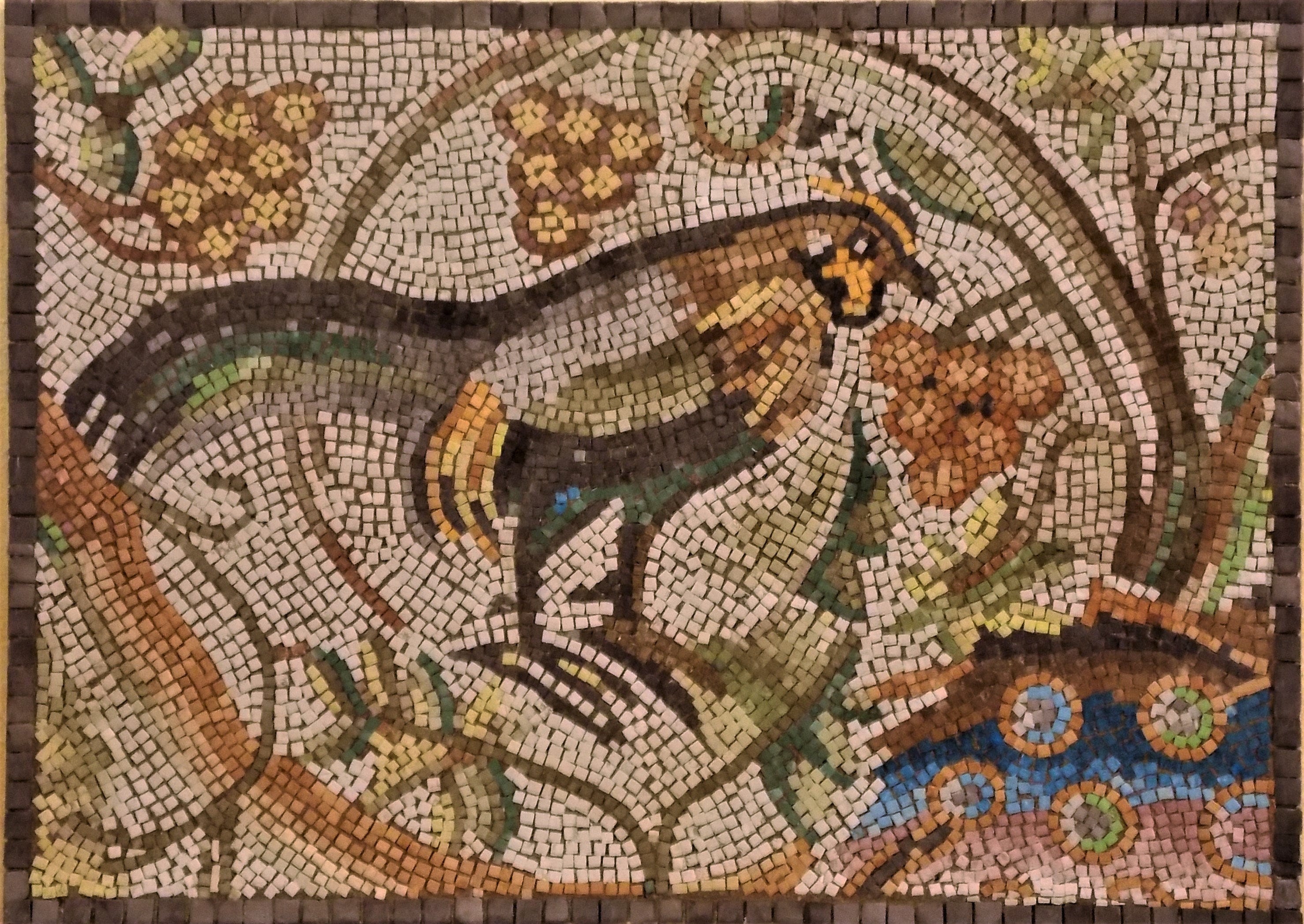This detailed stone mosaic artwork, comprised of thousands of vibrantly colored square tiles, intricately depicts a central image of a rooster standing upright and facing right. The rooster is vividly rendered in shades of black, white, brown, yellow, and even hints of green on the tail feathers, contributing to the detailed complexity of the piece. Surrounding the rooster, particularly in front beneath its head, is the face of a small, teddy bear-like figure, characterized by its brown color, large ears, black eyes, and black nose. 

Amidst the vibrant scene, the mosaic also features elements suggesting natural elements like tree branches, leaves, flowers, and possibly berries or cherries. These are subtly integrated throughout the background in various shades including greens, yellows, oranges, and tans. Unique to the lower right section, there's a concentration of blue tiles, forming a design that includes five concentric circles with a tan outer ring, which gives an impression of a colorful shell or a water element. Above this blue section, there’s a depiction of what could be a tree or vine shape. All these intricate details blend seamlessly against a predominantly white tile background. The entire mosaic is bordered by larger tiles in shades of tan and brown, enveloping the artwork and adding to its ornate frame.